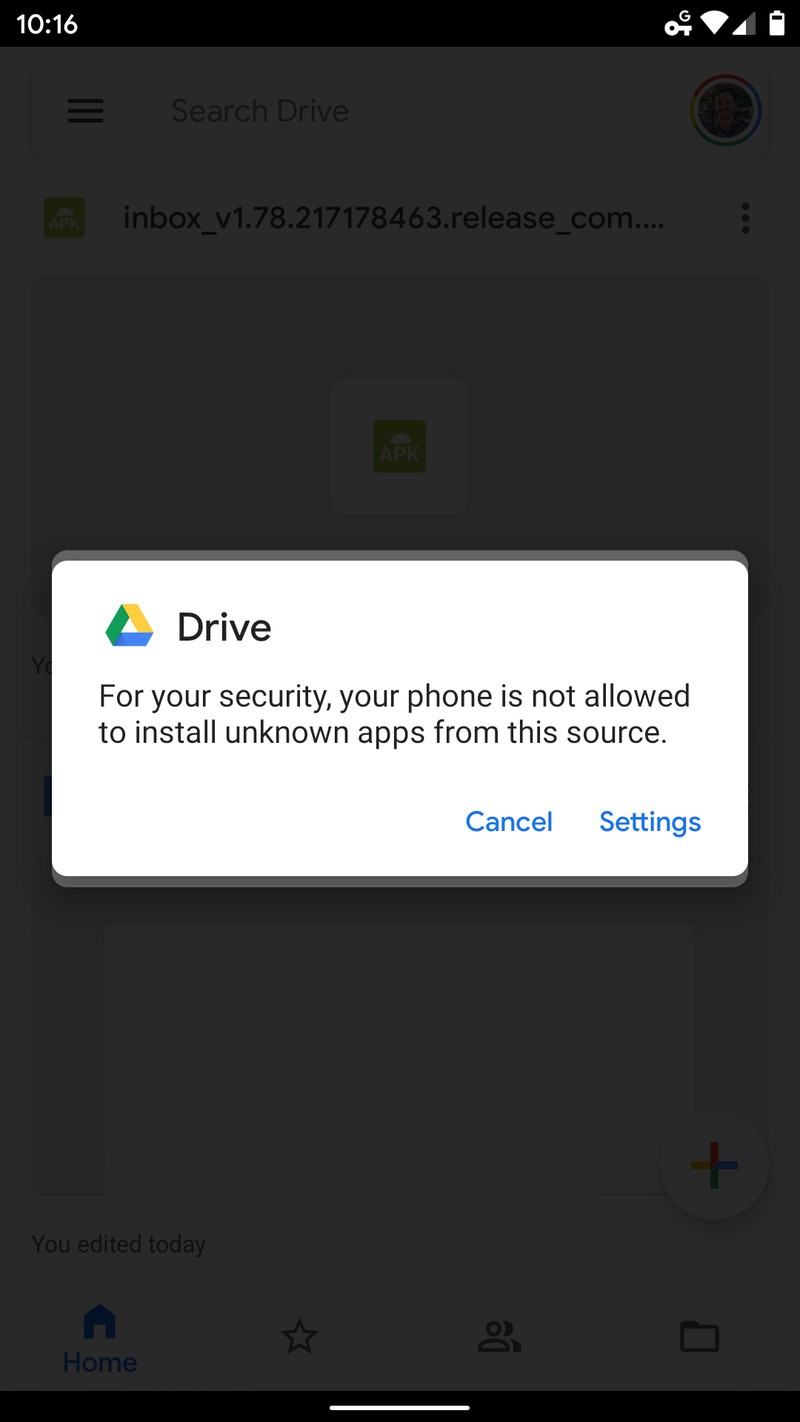This screenshot captures the Google Drive app interface on a cell phone. The primary focus of the image is a pop-up notification in the center of the screen. It features the Google Drive logo in the top left corner, accompanied by the word "Drive" in bold black letters. Below this, a security warning message reads: "For your security, your phone is not allowed to install unknown apps from this source." 

At the bottom of the pop-up, there are two small blue options: "Cancel" on the left and "Settings" on the right. The semi-transparent dark overlay background allows partial visibility of the underlying Google Drive home screen. At the very top, under the overlay, there's a search bar labeled "Search Drive," flanked by a user profile icon on the far right and a menu icon on the far left.

Immediately beneath this toolbar, a file listing is partially visible. The listing is displayed on a white rectangular bar and is identified by the name "Inbox" along with its corresponding file number. A small green icon is situated to the left of the file name, while a horizontal three-dot options icon is located to the right.